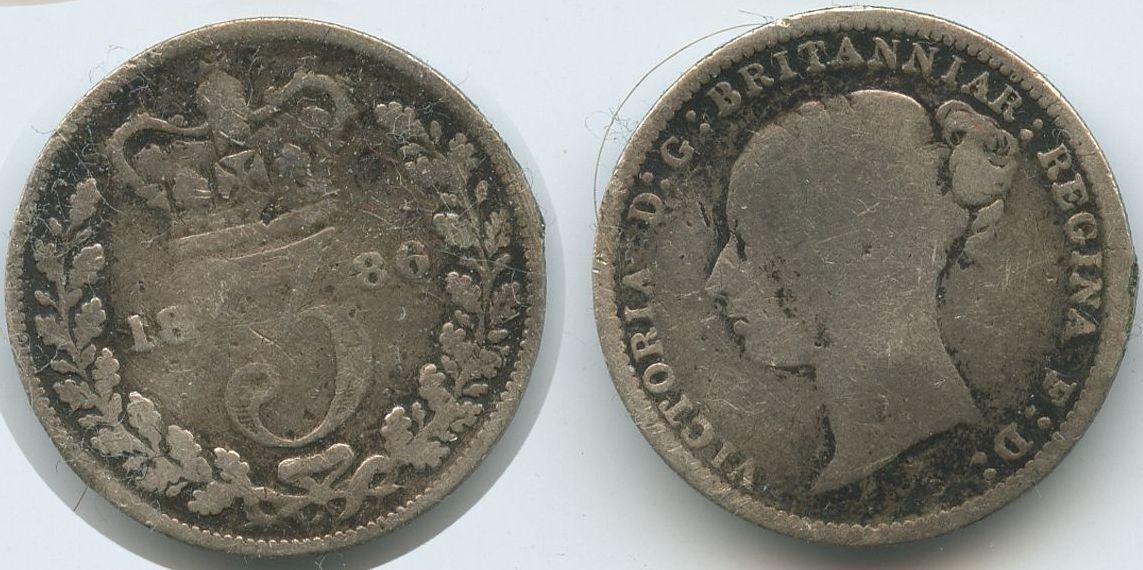The image displays two well-worn, weathered silver coins, likely showing the obverse and reverse sides of the same coin. On the left side, the reverse side of the coin features the year "1886" with "18" on the left and "86" on the right, surrounding a large, central number "3". At the top, there is a crown, and an olive-like wreath encircles the edge of the coin. On the right side, the obverse shows a woman's profile facing left, with her hair styled in a bun at the back of her head. Surrounding her image are the inscriptions "Victoria D.G. Britanniar Regina F.D." Although the coin is quite worn, the details remain distinguishable, depicting an era from Victoria's reign in 1886.